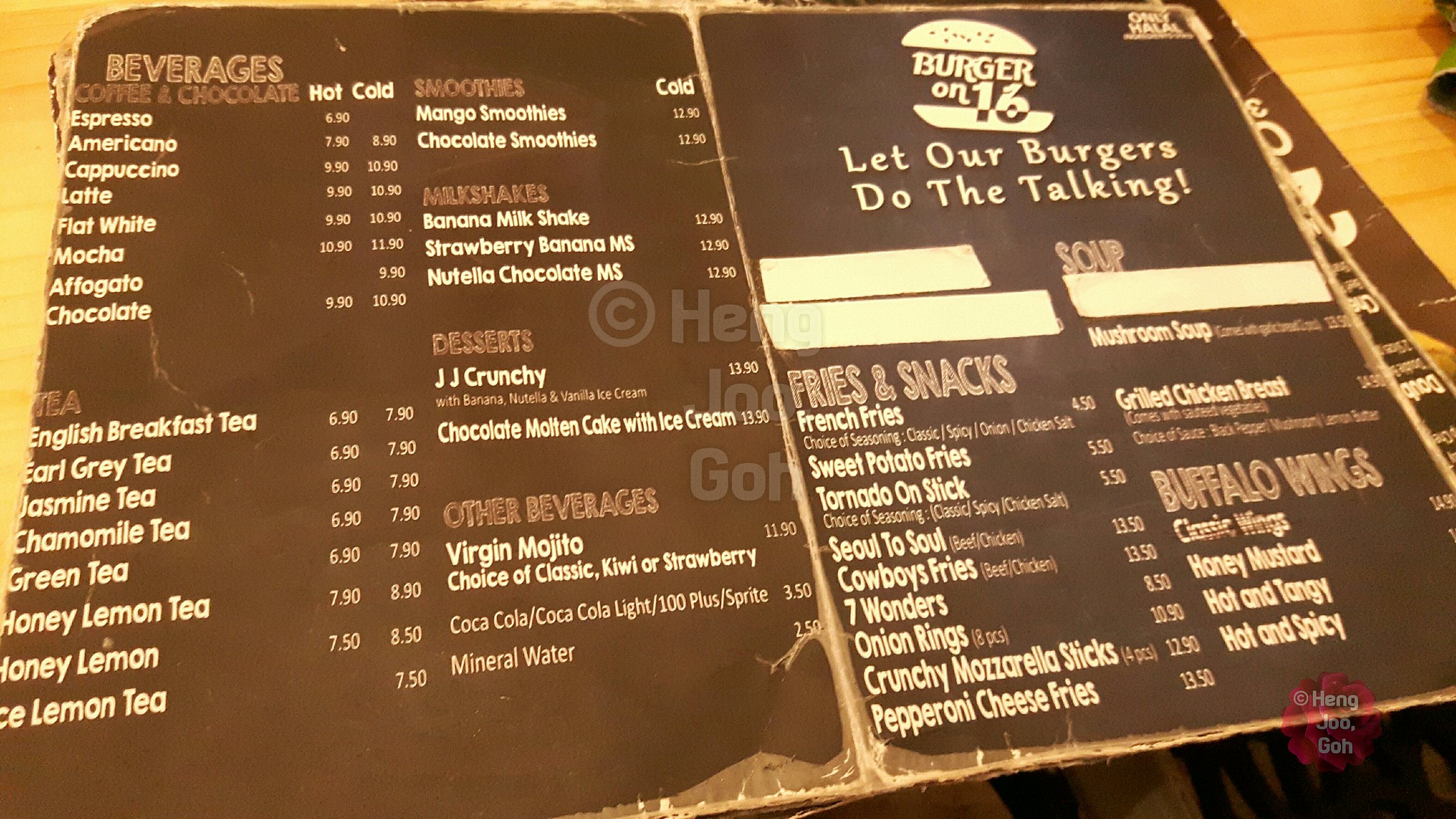This image features a worn and tattered restaurant menu displayed on a wooden table, captured in landscape orientation. The menu, predominantly blackish-brown, is divided into two segments with a noticeable white crease marking the fold. Its surface is heavily damaged, exhibiting numerous wrinkles, cuts, rips, and tears, reflecting its frequent use.

At the top section of the menu, a distinct orange headline reads "Beverages," followed by subcategories such as "Coffee and Chocolate" in a darker shade of orange. This section lists approximately seven drink options in white text. The middle part of the menu introduces another category labeled "Tea," presenting about eight selections.

Along the left margin, the menu features a white logo that reads "Burger on 16" accompanied by the tagline "Let our burgers do the talking." Adjacent to this are various columns: "Smoothies" with two choices, "Milkshakes" listing three, a column for "Desserts" with four options, and "Other Beverages" also offering four choices.

Additionally, a section titled "Fries and Snacks" appears halfway down the page, detailing several snack options, followed by a "Soup" category listing a few soups. Below this, there is a segment for "Buffalo Wings" offering various selections. Notably, the menu has two white rectangular areas, indicative of content being taped over or concealed, one above the "Fries and Snacks" section and another below the "Soup" section.

In the background, a faint watermark partially obscured by the menu starts with an 'H,' followed by another word beginning with an 'I' and concludes with a third word starting with a 'G,' though it is challenging to decipher due to insufficient contrast.